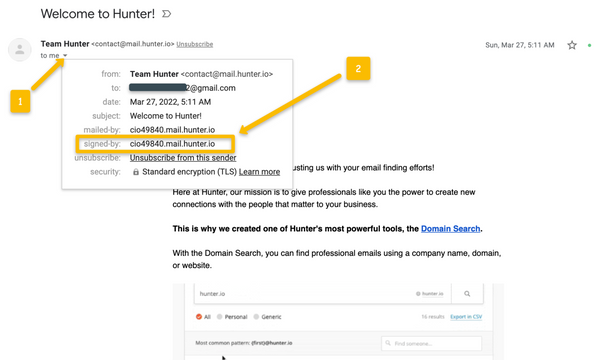In this image, we see a detailed view of a work-related website interface designed to facilitate team collaboration. The header at the top features an arrow labeled with the number '1' pointing to the text "Team Hunter" along with the contact email "gmail@hunter.lo." Below this, there's a message box displaying the following information: 

- From: Team Hunter
- To: [Recipient's email is blacked out]
- Date: March 27th, 2022, 5:11 a.m.
- Subject: Welcome to Hunter

The email contains metadata with fields such as "Mailed by," "Signed by," "Unsubscribe," and "Security: standard encryption, learn more." Another arrow labeled '2' points to the "Signed by" field, highlighting its significance.

Outside of this message box, although partially cut off, the text continues to promote Hunter's services. The visible part of the sentence reads: "...us with your email finding efforts here at Hunter. Our mission is to give professionals like you the power to create new connections with people that matter to your business." This content signifies that Hunter is a business-oriented platform.

A key feature highlighted in the email is "Hunter's most powerful tools, the domain search." The phrase "domain search" is hyperlinked and colored blue, indicating that it is clickable. The text elaborates: "With the domain search, you can find professional emails using a company name, domain name, or website." This further emphasizes that the website is a professional tool aimed at enhancing business networking and email discovery.